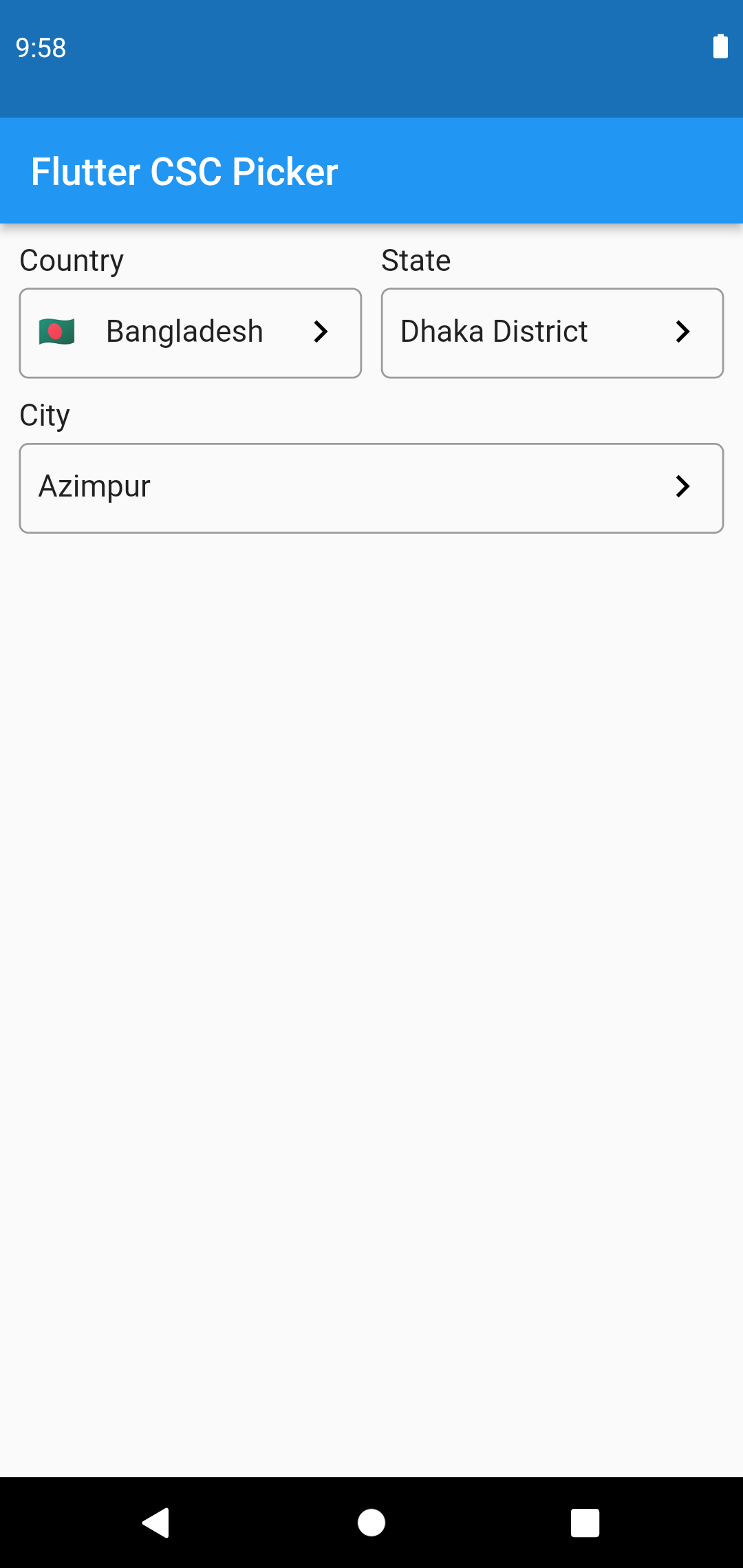The image is a vertical screenshot likely taken from a smartphone. At the very top, there is a navy blue rectangular box displaying the time "9:58" in white, accompanied by an unidentified white icon on the right side of the box. Below this, a lighter blue box contains the text "Flutter CSC picker" in white. Underneath this, the background shifts to a gray hue, and it displays selected location details: "Country: Bangladesh, State: Dhaka District, City: Azimpur." At the bottom of the screen, there is a long rectangular black navigation bar featuring three icons: a white triangle pointing left, a circle in the middle, and a square to the right.